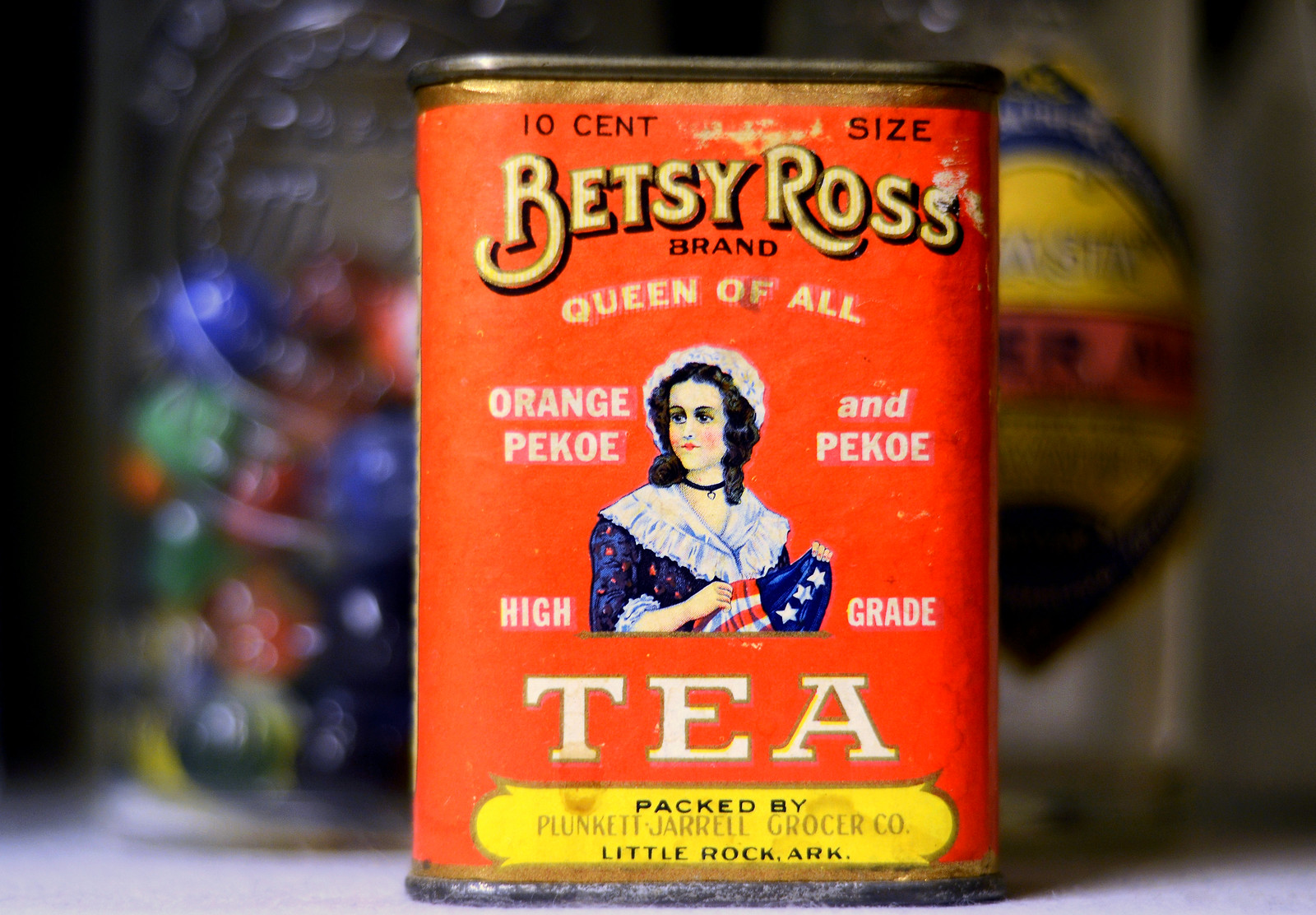This image depicts a small, square, vintage metal canister of tea against a painted orange background. The canister, which looks quite old, features gold lettering that reads, "Betsy Ross Brand, Queen of All, Orange Pekoe and Pekoe, High-Grade Tea." It also indicates a price of "10 cents" and notes the tea was packed by the Plunkett-Jarrell Grocer Co., based in Little Rock, Arkansas. The label showcases an illustration of Betsy Ross, the renowned figure from the American Revolutionary War credited with making the first U.S. flag. She is depicted with brown hair, red lips, wearing a bonnet and a frilly blue dress with a collar. In her hand, she holds an American flag. The overall style of the canister, from its design to the typography, exudes a distinctly vintage feel, further emphasizing its age and historical significance.